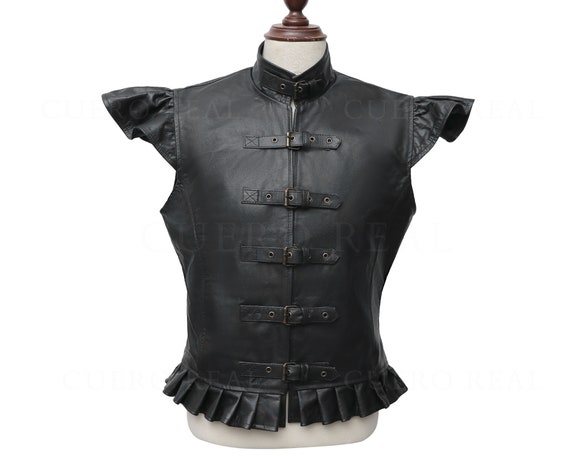The image depicts a white dressmaker's dummy in a bust format, lacking a head, arms, and lower half, and topped with a small wooden frame where the head would be. Displayed on the dummy is a vintage gothic black leather coat that combines features of both a vest and a jacket. The intricate design includes short sleeves with ruffled tops extending a few inches from the shoulders, and further ruffles around the waist. The front of the coat is fastened with five evenly spaced buckled straps, made of a brassy, bronzy metal, which overlay a zipper. The coat extends upwards into a high-neck style, resembling a turtleneck with an additional belt-like strap across the neck. This meticulously crafted piece, with its pleated bottom and prominent hardware, exudes an antique, gothic charm. The entire scene is detailed in stark colors of black, white, and touches of brown, contributing to its vintage appeal.